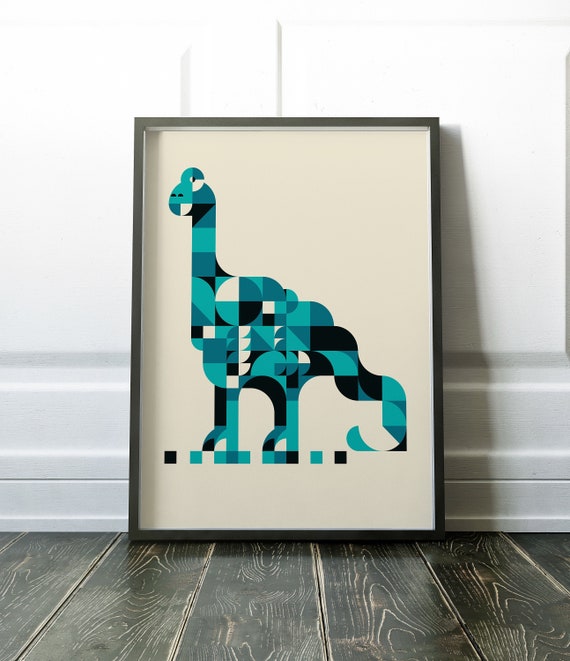This photograph captures a piece of framed artwork, set against a white wall and positioned on a dark walnut-hued hardwood floor, characterized by prominent wood grain lines. The black frame houses an abstract representation of a Brontosaurus, depicted in a side profile with its head on the left and tail curving to the right. The dinosaur's design is a patchwork of geometric shapes, particularly triangles, squares, and segmented circles. The prominent circular motif near the base of its neck is divided into four segments, featuring shades of dark green, light green, black, and white. The dinosaur’s legs, resembling stacked Lego blocks, are also green and squared off. Dominated by a palette of greens, blacks, and whites, the artwork's detailed textures create a pixelated effect, contributing to its unique and intricate appearance. The scene is completed by the artwork being leaned casually against a sturdy white cabinet.